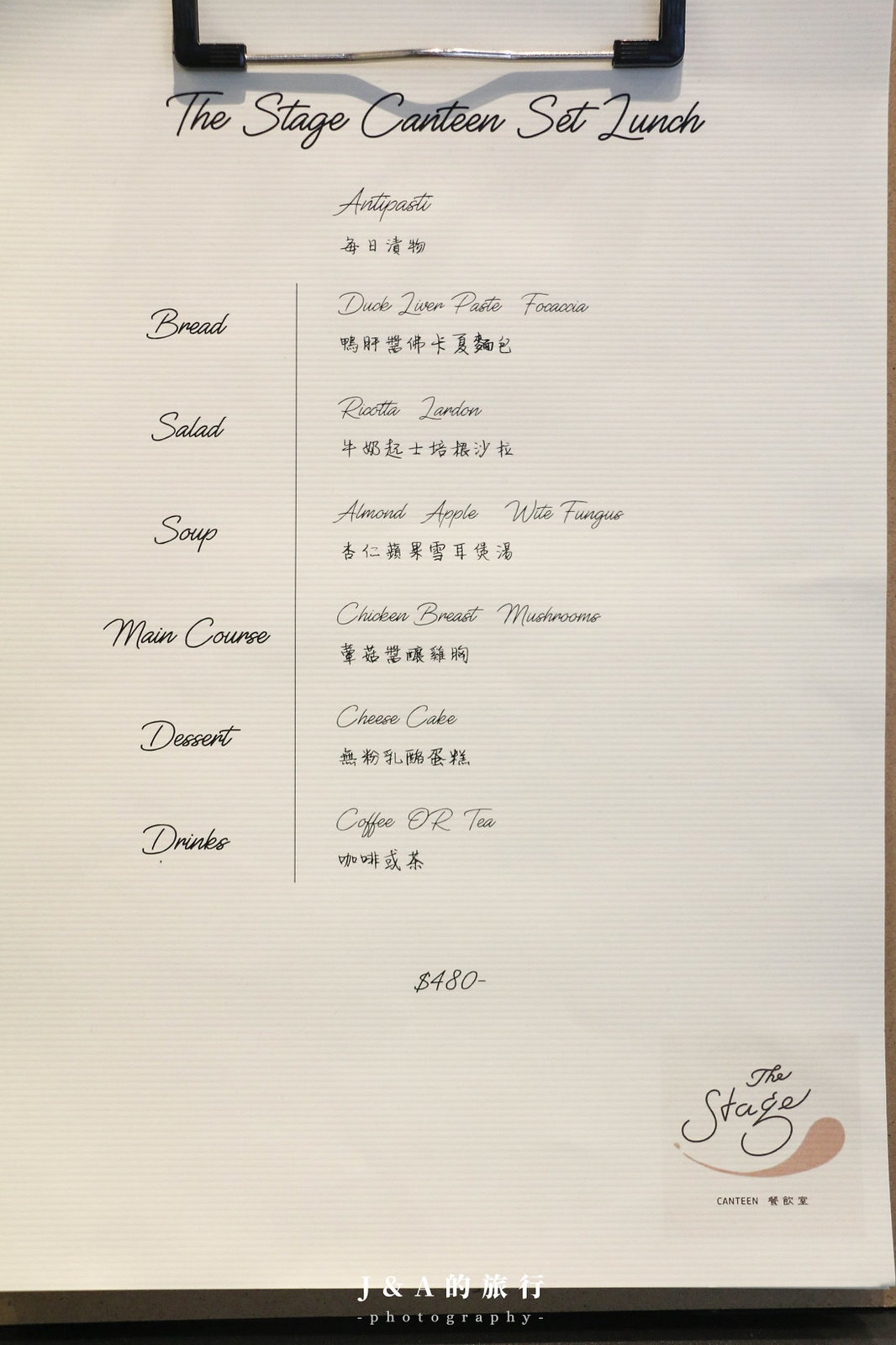The image showcases a meticulously crafted mock-up of a set lunch menu for "The Stage Canteen." This bilingual menu features both English text and Asian characters, adding a touch of cultural diversity. At the top, the menu is titled "The Stage Canteen Set Lunch," indicating its special offering. A matching logo, inscribed "The Stage Canteen," is positioned in the bottom right, confirming the restaurant's name.

The menu is sectioned into categories listed in the left column: bread, salad, soup, main course, dessert, and drinks. The corresponding dishes are as follows:

- Bread: Duck Liver Pate Focaccia
- Salad: Risotto London
- Soup: Almond Apple White Fungus
- Main Course: Chicken Breast with Mushrooms
- Dessert: Cheesecake
- Drinks: Coffee or Tea

A notable detail is the price, set at a premium $480 USD. Presented on parchment-like paper and secured to a clipboard, the menu exudes a rustic yet elegant aesthetic. A subtle watermark at the bottom, marked "J&A Photography," suggests the involvement of professional photographers in creating this refined mock-up. The overall presentation hints that this is a conceptual design rather than an actual photograph of a real menu.